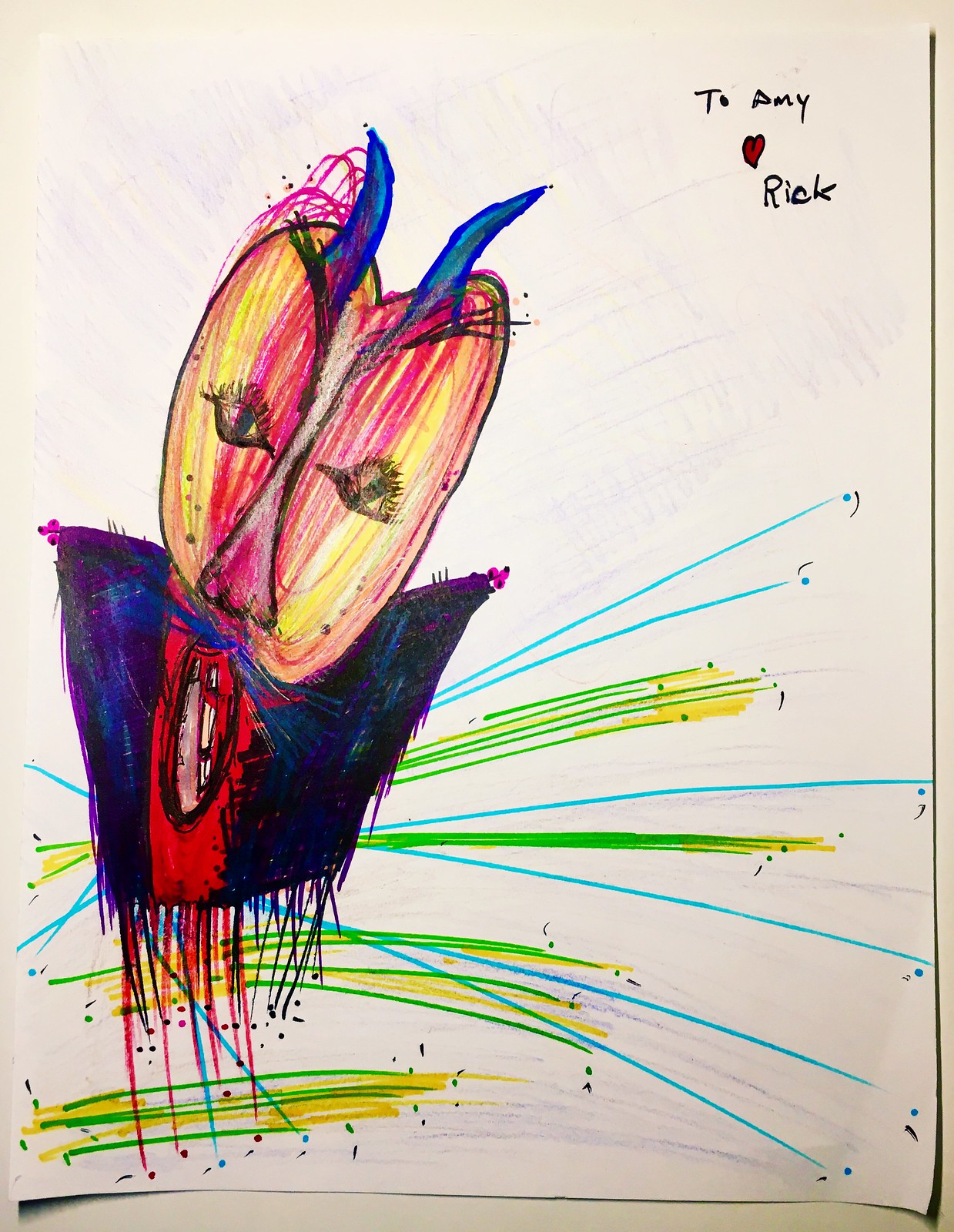At the very top of the image, there’s a white piece of paper with the word “aiming” written on it. Below this, a small red heart outlined in black is centrally placed. Near the bottom, text is also present. In the bottom left corner, light blue, green, and yellow lines crisscross erratically, giving a scratchy effect. On the far left side of the image, there's a figure depicted. The individual appears to be extending both arms, as if they are holding a ping pong paddle in each hand. The figure’s torso features an open black square, and surrounding this are red splotches along with red, black, and blue lines. The eyes are drawn open and are detailed with noticeable eyelashes. The figure possesses a large, central nose. Blue hues accent the top left and right sections near the forehead, resembling horns, while purple shades and black highlights frame the rest of the face.